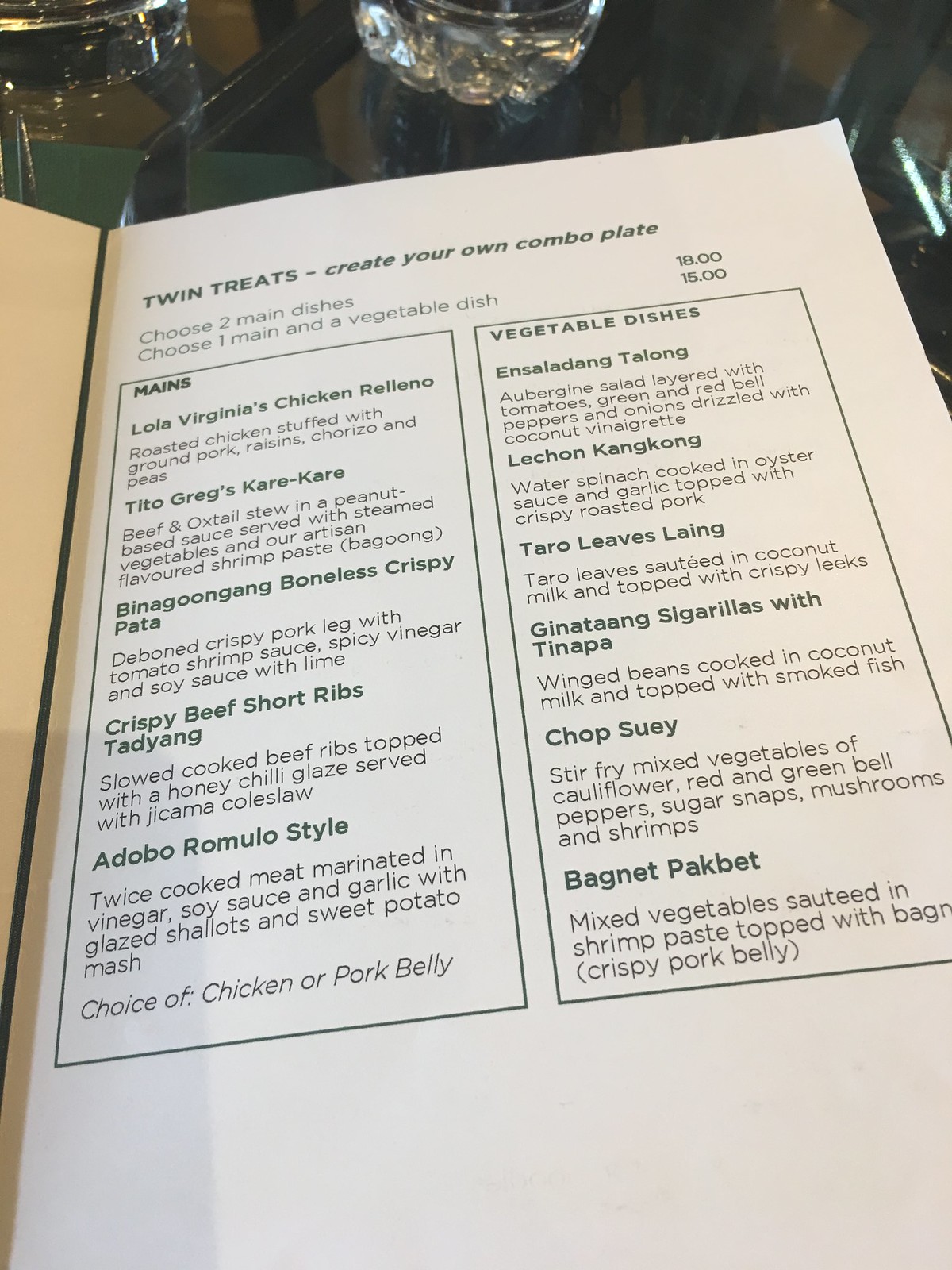This image shows a photo of a single page from a restaurant menu titled "Twin Treats, Create Your Own Combo Plate." The menu offers options to choose two main dishes for $18 or one main dish and a vegetable dish for $15. The left side lists the mains, including Lola Virginia's Chicken Relleno, Tito Greg's Kare-Kare, Bina Goongang Boneless Crispy Pata, Crispy Beef Short Ribs, Tadjang, and Adobo Romulo Style, with a choice of chicken or pork belly. The right side features vegetable dishes such as Ensaladang Talong, Lechon Kangkong, Taro Leaves Lang, Dina Tang, Sigarilla Swiss Tinapa, Chop Suey, and Bagnet Pak Bet, which consists of mixed vegetables sautéed in shrimp paste topped with crispy pork belly. There is a glass visible near the menu, adding a touch of real-world context to the setting. The menu page appears to convey traditional Filipino cuisine with creative and hearty dishes.